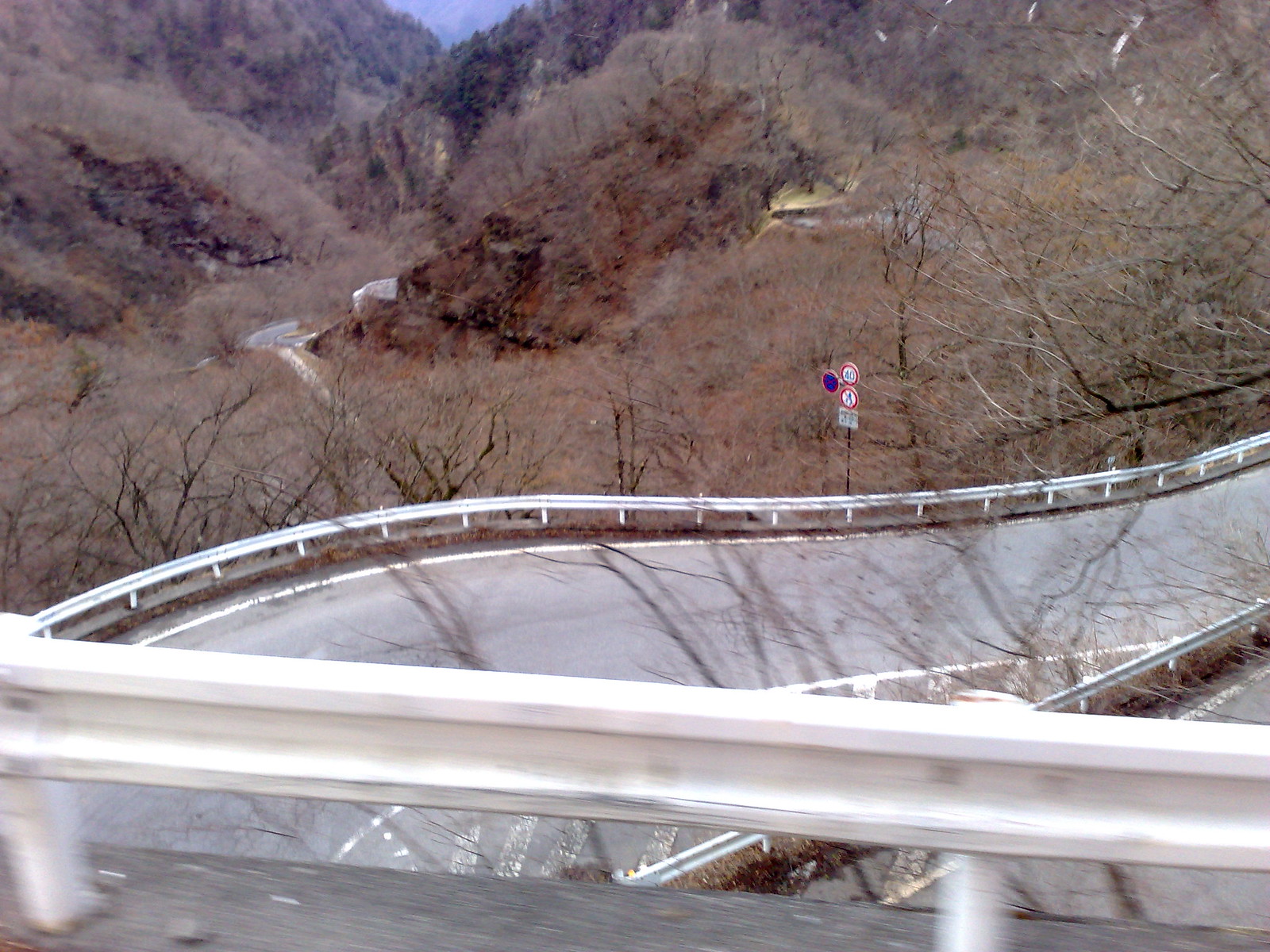The photograph features a winding road high in a mountainous region, captured from behind a metal crash barrier that extends horizontally across the bottom foreground. The guardrail, typical of those found on roads, highways, or mountain passes, is slightly blurred, adding depth to the image. The road itself starts in the bottom left corner, winding off into the distance towards the center right of the image. It has an undulating surface and a noticeable bank angle on the left side, suggesting it could be a racing or test track rather than a public road.

In the middle ground, to the left of the road, stands a black pole with a triangular arrangement of three circles—one blue and red circle on the left, a numbered circle on the upper right, presumably indicating a speed limit of 40, and another sign at the bottom left. There are no vehicles present on the road, which is made of grey asphalt and marked with a white line along its left edge.

The background features a rugged landscape with steep mountains rising on the left and a ridge extending out of the frame to the right. The terrain is dotted with barren bushes, twigs, and large grey and brown rock formations, devoid of any greenery. The overall scene is stark and desolate, highlighted by leafless trees and patches of dead grass, emphasizing the harshness of the environment.